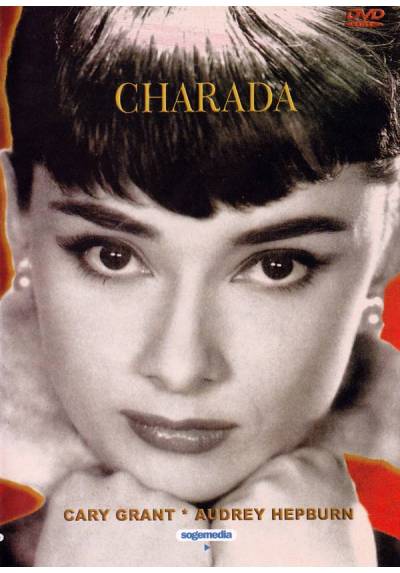The image is a vintage-style DVD cover featuring a close-up of Audrey Hepburn. The title "CHARADA" is prominently written across the top in a goldish-yellow, capitalized font, integrated into her dark, short-cut hair. Audrey’s big eyes and thick dark eyebrows stand out as she gazes straight ahead with a neutral expression, her hands gently placed under her chin. She appears to be wearing pearl earrings. The background has subtle hues of red. At the bottom, over her knuckles, the names Cary Grant and Audrey Hepburn are displayed with a bullet point separating them, also in goldish font. Beneath their names, the small blue text reads "SOGMEDIA," accompanied by a little blue play emblem. The top right corner of the cover includes a small red DVD logo.